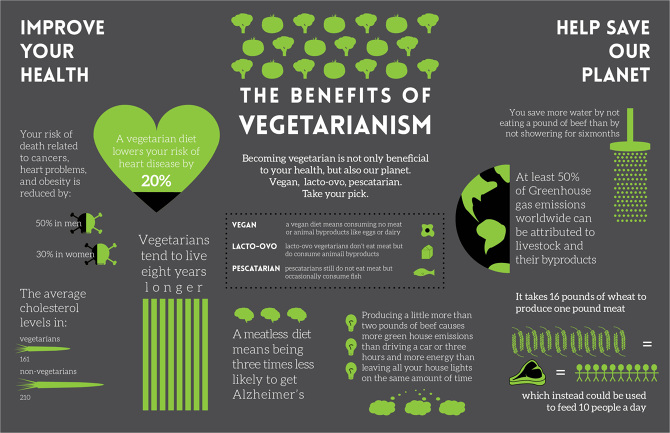This image depicts a gray sign covered in text and images promoting the benefits of various vegetarian diets. At the top of the sign, green images resembling vegetables such as broccoli, cauliflower, and tomatoes provide a colorful border. 

The upper-left corner features the phrase "Improve your health" in white letters, emphasizing health benefits. Nearby, it details how a vegetarian diet reduces the risk of death related to cancers, heart problems, and obesity by 50% in men and 30% in women. Additionally, it states that such a diet lowers the risk of heart disease by 20% and suggests vegetarians tend to live eight years longer, thus extending their lifespan into their 80s.

On the upper-right, another callout in white letters reads "Help save our planet," underlining the environmental advantages of adopting vegetarianism. Supporting this claim, the poster mentions that at least 50% of global greenhouse gas emissions can be attributed to livestock and their byproducts.

Central to the sign, large white letters proclaim "The Benefits of Vegetarianism," followed by smaller text explaining that choosing a vegetarian lifestyle is beneficial not only for personal health but also for the environment. The sign encourages readers to consider various diet options such as vegan, lacto-ovo, and pescetarian, and a small black rectangle at the bottom provides definitions for these terms.

Interspersed around the sign are additional green images and white text reinforcing the health and environmental benefits, including a note that a meatless diet makes one three times less likely to develop Alzheimer's disease.